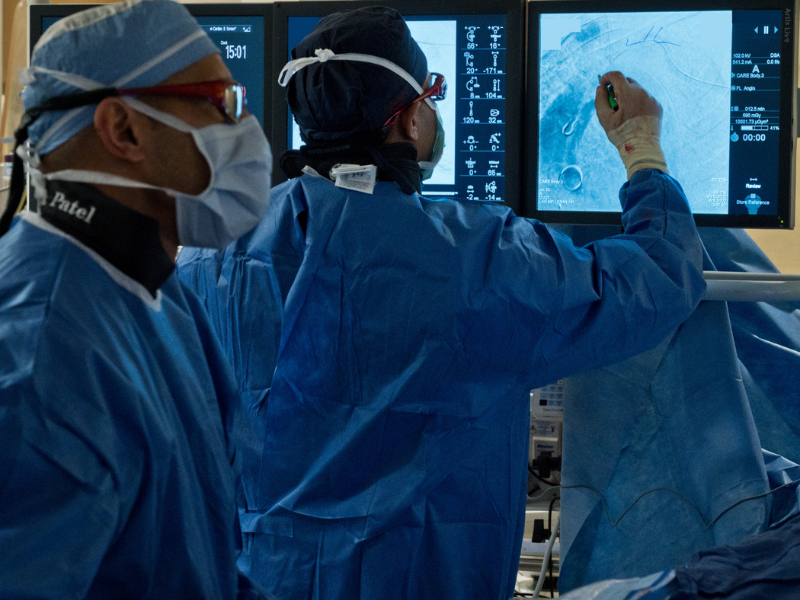In this detailed indoor photograph, two medical professionals, likely surgeons, are captured in an operating room setting. Both are adorned in blue surgical gowns, white face masks, blue head caps, and eyeglasses. The doctor on the left is in profile, with a neckband displaying the name "Patel." His colleague stands with his back to the camera, closely examining a monitor. This second doctor is pointing at a blue-tinted screen with his right hand, holding what appears to be a marking utensil. There are two screens visible; the one on the left shows a series of complex numerical markings including 50, 16, 20, -17, and 104. The right screen, identified by the text "August, C-A-R-E, 0-1-2-5-M-I-N" at the top right corner, appears to be displaying an x-ray image of a body. In the bottom right corner of the image, there's a glimpse of a blue blanket or towel. The scene reflects the surgeons' focused collaboration, presumably in the midst of a critical medical procedure.